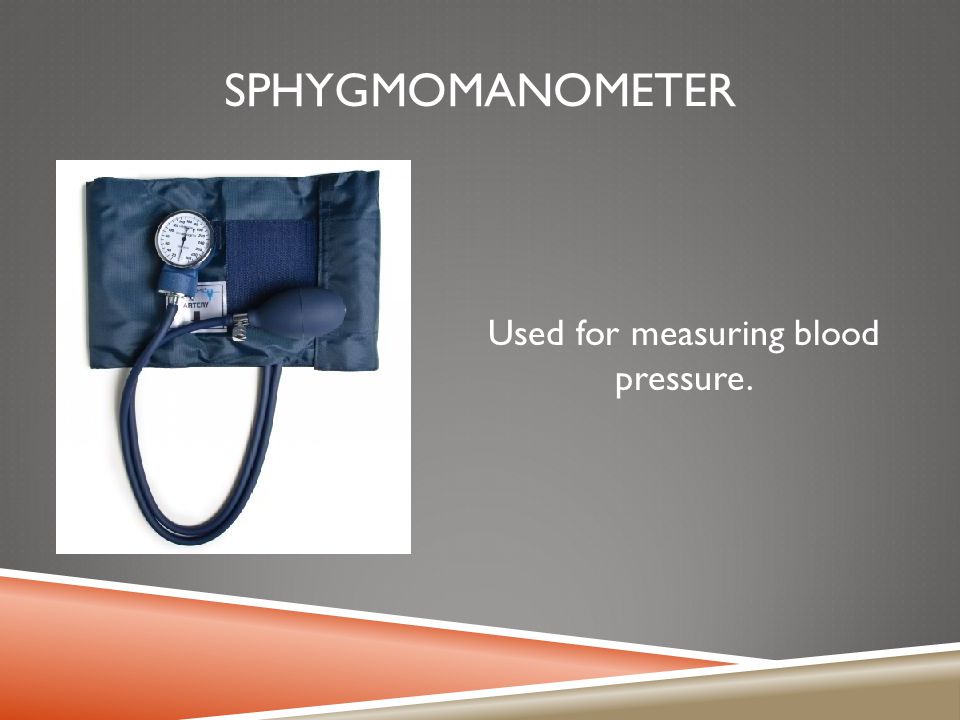The image showcases a sphygmomanometer, prominently labeled at the top in white text as "sphygmomanometer." The depicted medical device, used for measuring blood pressure, is navy blue in color and consists of several components: a cuff, a squeezable bulb, and a circular dial that resembles a clock face. This dial, featuring a white interface with numerical indicators, is essential for reading blood pressure levels. A navy blue tube connects the cuff to the bulb. The background of the advertisement is predominantly gray, accented by diagonal lines of pink and tan at the bottom. Additionally, the right side of the image bears the explanatory text "used for measuring blood pressure."